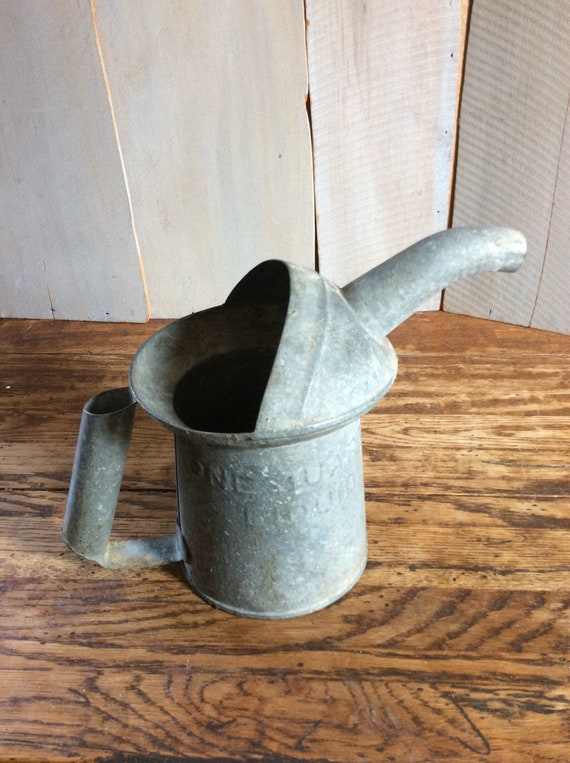The photograph showcases an old, weathered metal oil can or watering can with a dull gray, oxidized finish. It features a cylindrical hollow handle on the left and a spout on the right, emerging from a partially covered top. The can’s circular base rests on a worn, dark-grained wooden table. Imprinted on the side of the can are indistinct impressions or characters, suggesting old usage. The background consists of vertical white wooden slats, adding to the rustic atmosphere. The inside of the can is notably dark, with a black center where liquid would be poured. Its appearance and setting evoke a sense of antiquity and rugged utility.